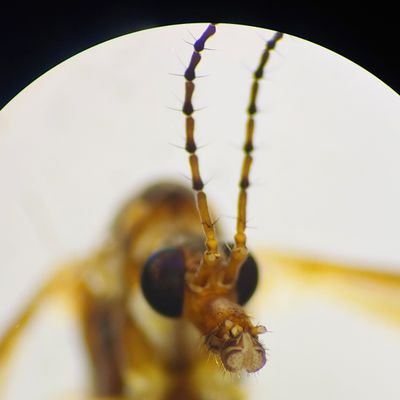This striking close-up photograph features the head of a bright yellow-brown insect, showcasing intricate details of its facial structure. Dominating the image are the insect's two large, round black eyes, each occupying nearly half of its tiny head. A long, protruding snout extends from the center, flanked by two straight antennae featuring black-tipped segments with tiny hairs visible on either side. The sharply focused head contrasts with the blurred golden-brown wings and darker legs, hinting at the insect's capacity to fly. The surrounding backdrop features a partial white circle against a black background, adding depth to the composition while enhancing the insect's vivid colors and defining its form.